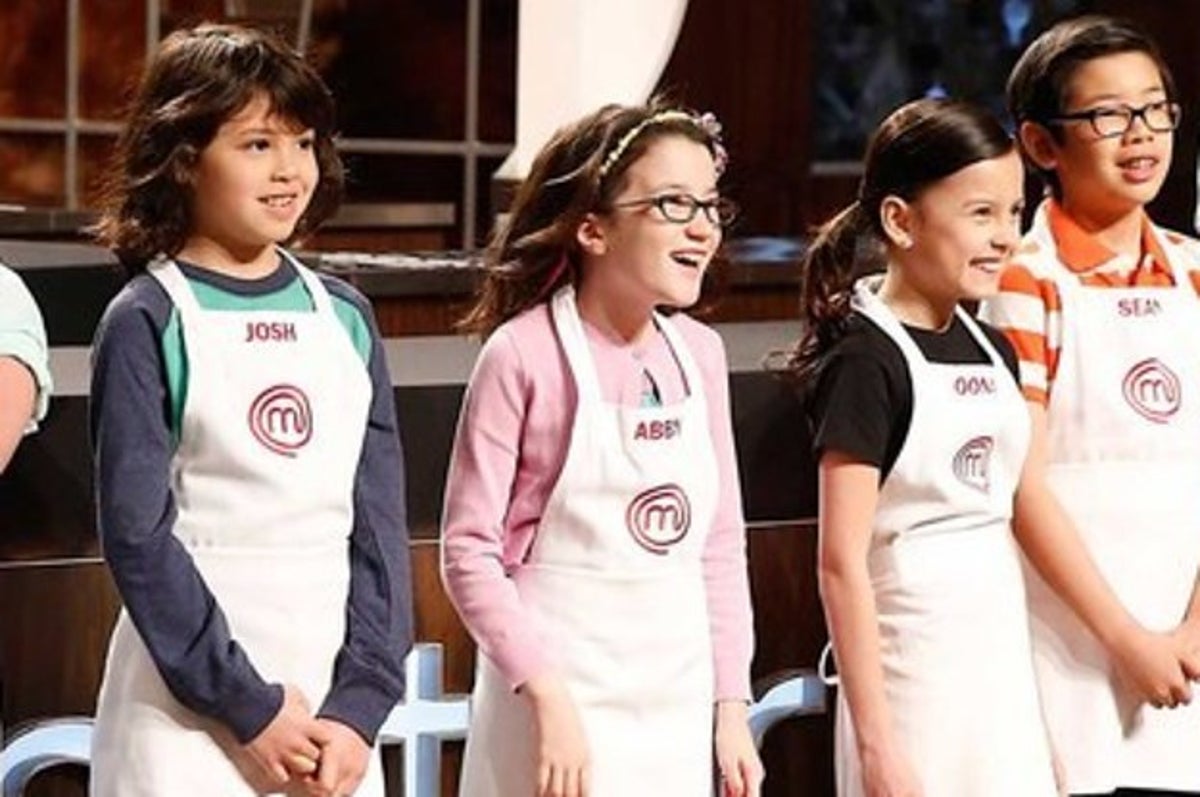The image depicts a cheerful group of four young children, presumably participating in a cooking contest similar to MasterChef. They're standing in a kitchen setting, with visible countertops and stovetops in the background. Each child wears a white apron emblazoned with their name. From left to right: the first child, Josh, has long hair; next to him is Abby, who is wearing glasses and a pink shirt; the third child, dressed in a black t-shirt, has an indistinct name, possibly "Uno"; and the last child, Sean, also wears glasses and a white and orange striped shirt. All the children are smiling, contributing to the happy and enthusiastic atmosphere of the scene.